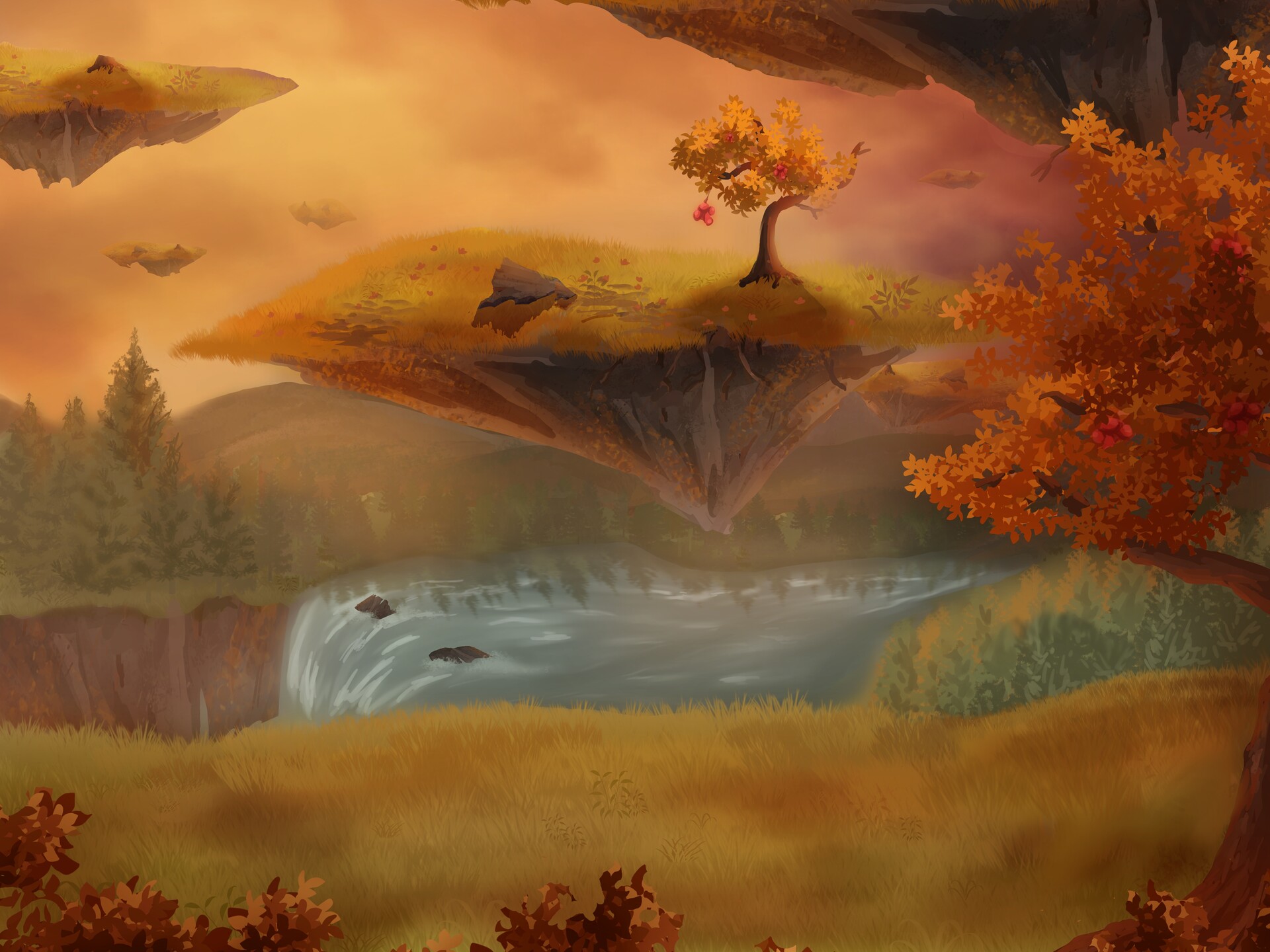The painting vividly captures a fantastical, almost magical landscape with multiple floating islands seemingly torn from the earth. The scene is dominated by a waterfall at the center, where a river flows off the edge of a light green-brown grassy terrain. The bottom of the painting features some scattered leaves, mainly brown, transitioning to grassy areas that stretch across from right to left. 

In the middle, there's a significant floating island hovering above the waterfall. This island has a pointed shape at the bottom, as if forcibly removed from the ground, revealing roots and earthy textures. It is topped with yellowish-brown grass and home to a single, small tree adorned with yellow and brown oak leaves. 

The top left of the painting features another similar floating island with grassy and earthy textures, while the top right corner shows the underside of an additional landpiece with a mix of yellow and pink hues.

The sky above is a blend of cloudy gray tones interspersed with striking yellow, pink, and purple shades, adding to the painting’s ethereal quality. More orange and brown tree leaves are visible on the right side, contrasting against the vivid, surreal sky. This intricate detailing combines to create a scene that is both otherworldly and captivating.